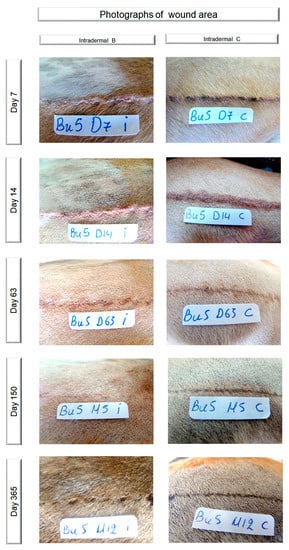The image is a detailed medical chart featuring 10 photographs that document the healing process of an incision over time. The chart is organized into two columns and five rows, with each row representing a specific time point: Day 7, Day 14, Day 63, Day 150, and Day 365. Along the left side, the timeline is labeled from top to bottom, showing the progression from initial incision to almost fully healed scar. Each column contains two photographs, depicting the wound at various stages of healing. The top of the chart includes black text reading "Photographs of One Wound Area," followed by the labels "Intradermal B" and "Intradermal C." The incisions, marked with identifiers such as "BU5D7I" and "D14I," appear to be on animals with fur, indicating the subject of the medical study. The photographs detail the transformation of the incision, starting from a fresh, rough-looking wound to a nearly invisible scar by Day 365.